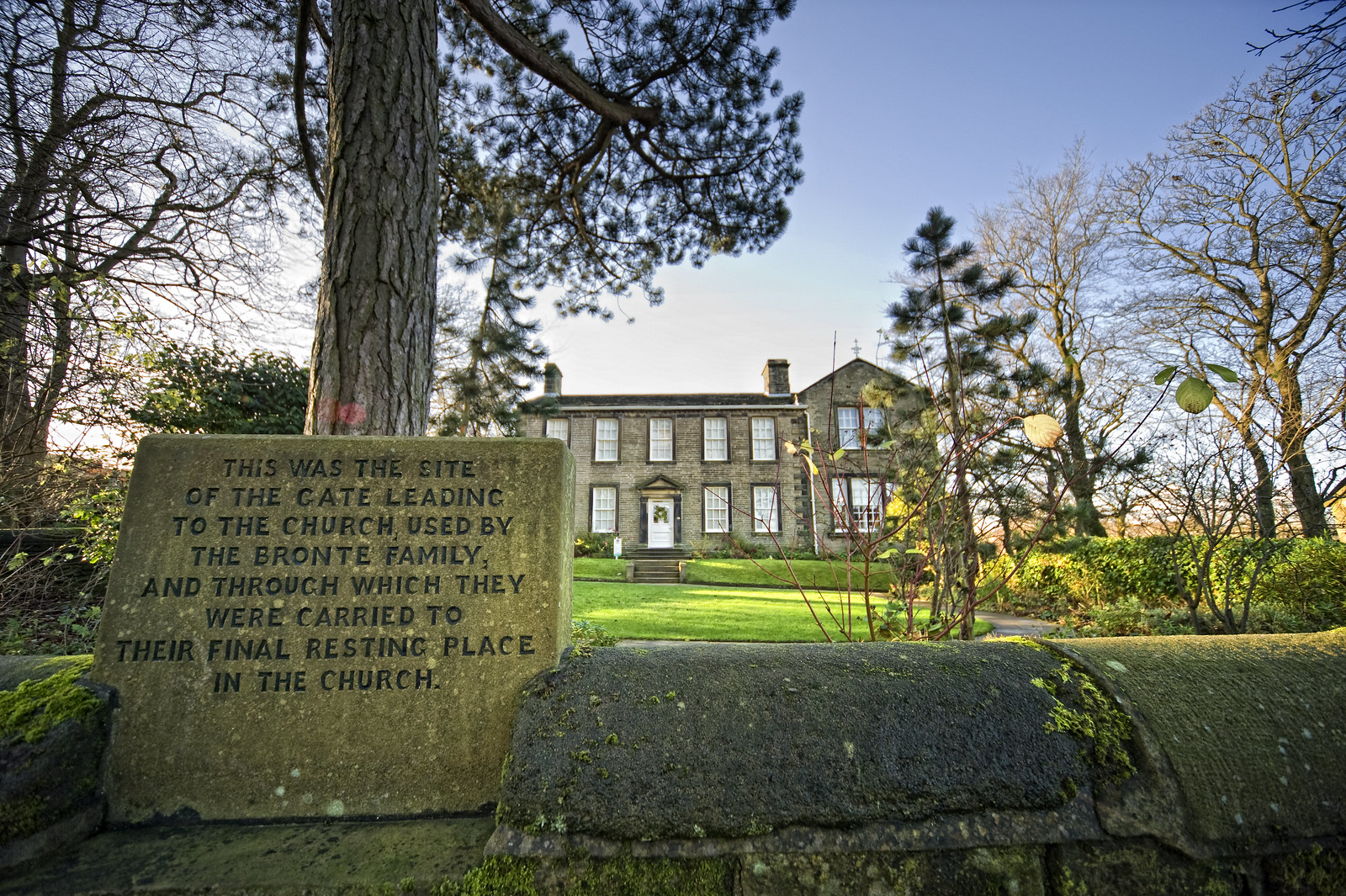In this photograph, a large historic stone house, the focal point of the image, stands in the middle distance. Its weathered gray stone façade showcases a white door with little stone steps leading up to it, and it is crowned by two stone chimneys, one on the near right and the other on the far left. The house is surrounded by a winter scene, with bare deciduous trees and evergreen pines, contributing to a serene, somewhat hazy atmosphere under a vividly blue sky that becomes misty near the horizon.

In the foreground, an old, smooth-topped stone wall, covered in patches of moss, stretches horizontally. Beside this wall stands a prominent brick plaque, about five feet tall, bearing an etched inscription that reads: "This was the site of the gate leading to the church used by the Bronte family and through which they were carried to their final resting place in the church." Just behind the plaque, a mature oak tree rises majestically, while neatly manicured grounds extend around the property, and other trees frame the view on the left and right, enhancing the historic and tranquil ambiance of the scene.